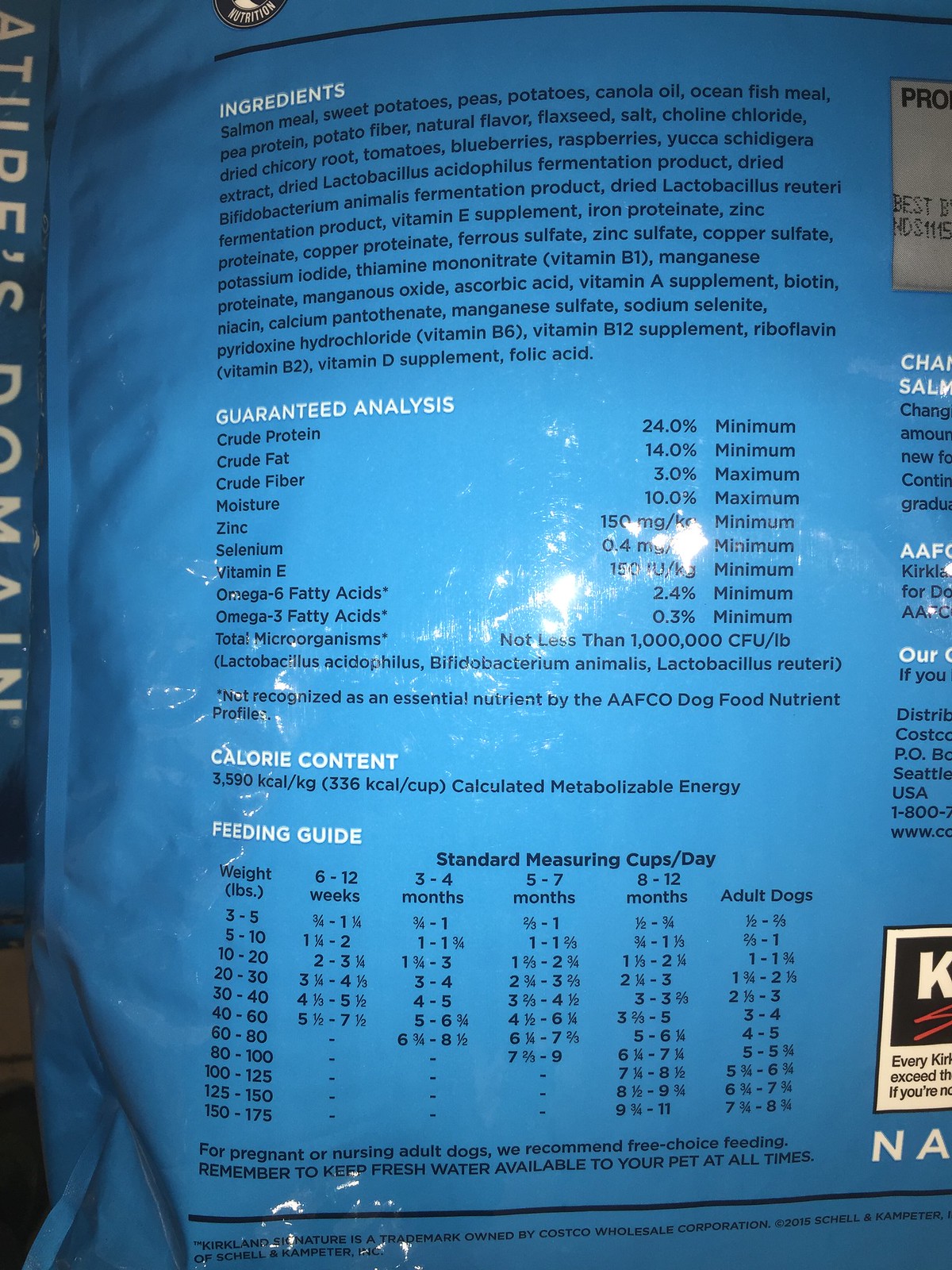The image shows the back of a blue dog food package, leaning towards a sky blue shade. The packaging prominently features sections written in white capital letters. At the top, it says "Ingredients" followed by a detailed list including salmon meal, sweet potatoes, peas, potatoes, canola oil, ocean fish meal, pea protein, potato fiber, natural flavor, flaxseed, salt, choline chloride, dried chicory root, tomatoes, blueberries, raspberries, zinc, and lactobacillus acidophilus fermentation product, among others. Below this, another section labeled "Guaranteed Analysis" breaks down the nutritional content, listing crude protein, crude fat, crude fiber, moisture, zinc, selenium, vitamin E, omega-6 fatty acids, omega-3 fatty acids, and total microorganisms, also noting that some nutrients are not recognized as essential by the AAFCO dog food nutrient profile. Further down, there are sections for calorie content and feeding guide, detailing the recommended daily feeding amounts based on dog weight, typically measured in standard measuring cups. The packaging also features a "Best By" date in black text on a white background and a partial view of the Kirkland logo with a red zigzag line. Additionally, there is a notice regarding care for pregnant or nursing dogs, advising to ensure fresh water availability.